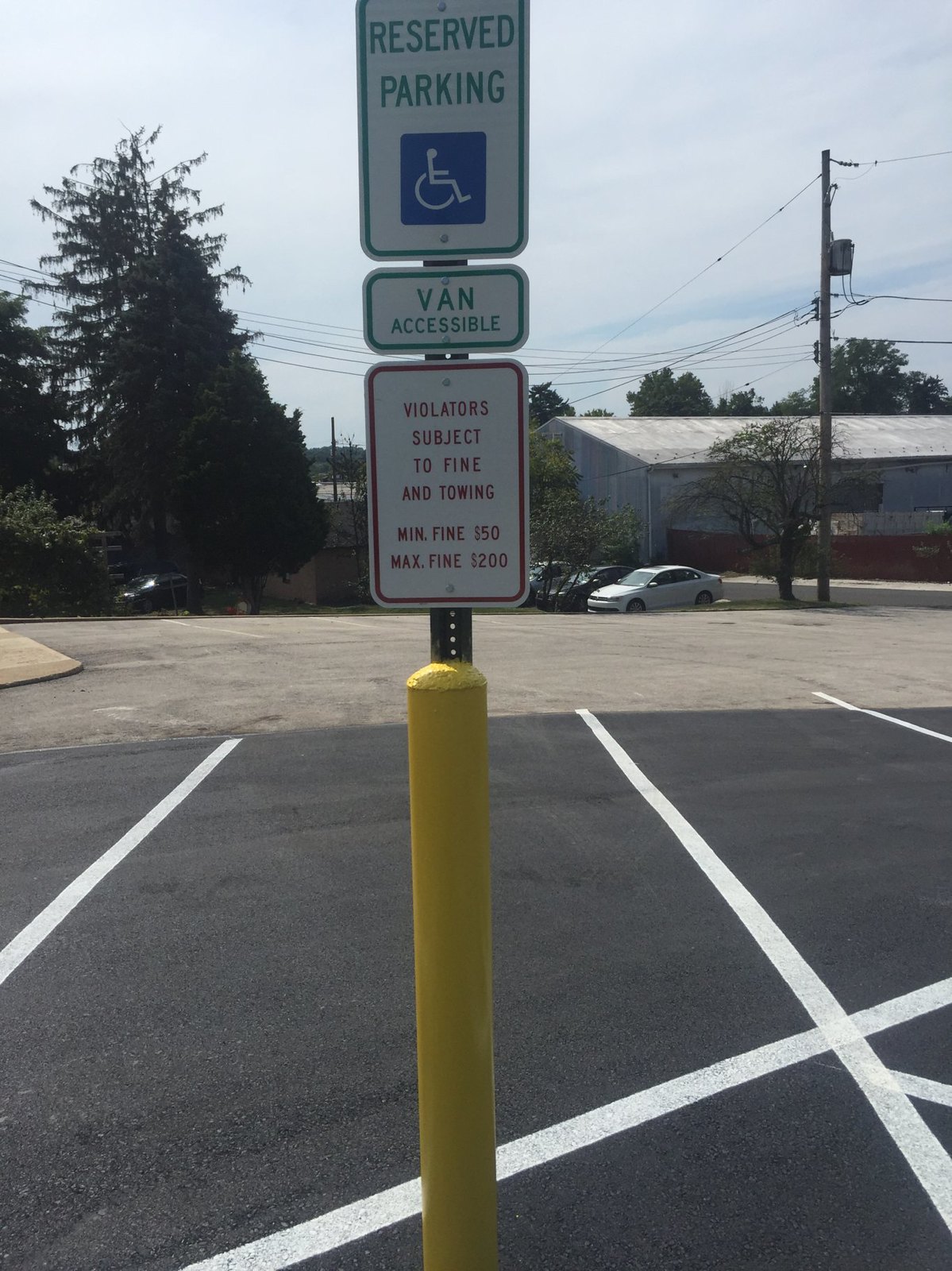The image depicts an outdoor daytime scene in a parking lot. Central to the image, a yellow pole about six to seven feet tall stands prominently, featuring a three-layered sign. The top plate has a green "Reserved Parking" text accompanied by a blue square containing the white wheelchair symbol, designating the spot as a handicap space. Directly beneath this, another sign with green lettering reads "Van Accessible." The bottom plate, bordered in red, warns that "Violators are subject to fine and towing" with fines ranging from a minimum of $50 to a maximum of $1200. The parking lot, with its crisp white lines marking the spaces, also contains a few parked cars. In the background to the right, a long metal shed extends across the width of the photograph, while a tall telephone pole and a large pine tree appear on the left, accompanied by several other trees.